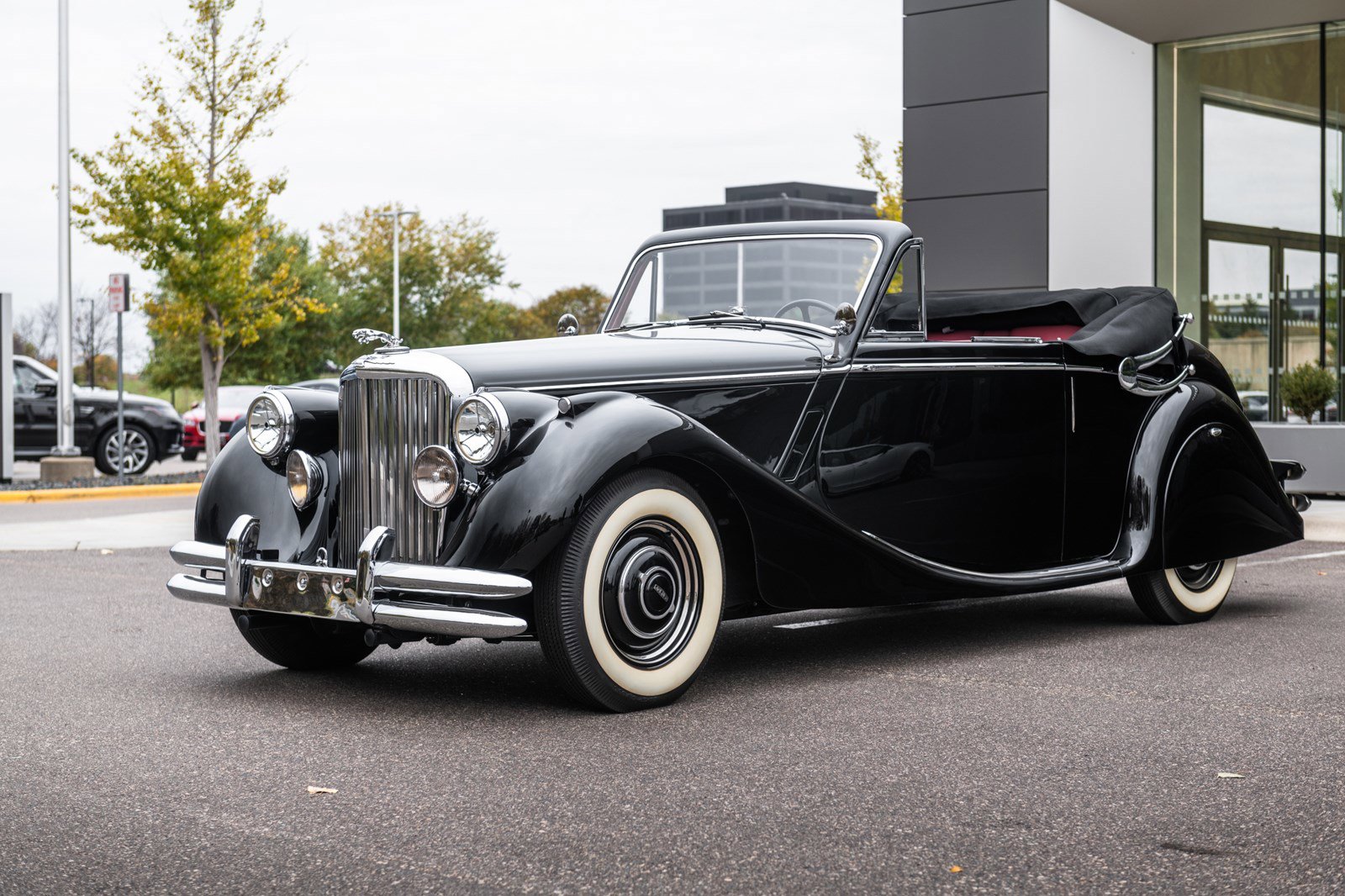A close-up shot captures a meticulously maintained black vintage convertible, likely from the 1920s or early 1930s. The car, resembling a Jaguar, gleams with its shiny black body and chrome details, including an elegant grille and robust bumpers. Four classic circular headlights, encased in stainless steel, adorn the front. The pristine white-walled tires contrast sharply with the black exterior, adding a touch of elegance. The hood is down, revealing black leather trim around the edges, and the interior appears to feature two seats. The backdrop includes a building with large windows, possibly a car dealership, situated on a tar-like surface. Through the windshield, more buildings and some signs are visible, along with parked cars and a thoroughfare. The sky above is white and slightly hazy, while trees punctuate the scene, adding a touch of natural greenery to the urban setting.